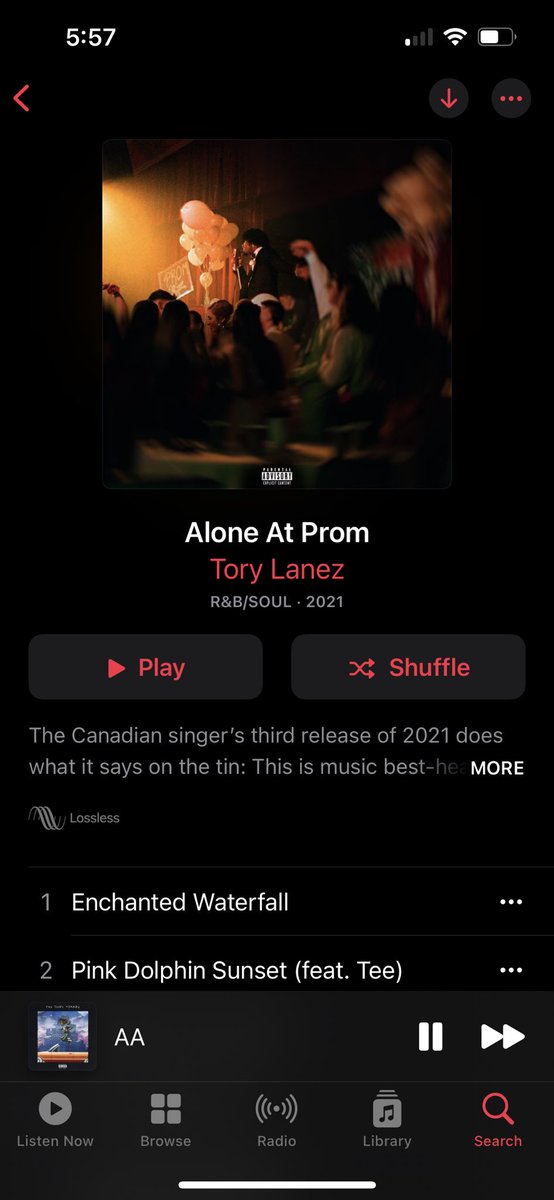The image depicts a music playlist on a platform that is likely not Spotify, possibly an app named Lossless, indicated by an emblem featuring three wavy lines above the song title that says "Lossless." The interface details such as the play, shuffle, and search buttons, as well as the artist's name "Tori Lannes," are all highlighted in red. Positioned at the top of the screen, the time reads 5:57, showing a network signal with one out of four bars, full Wi-Fi, and a battery level slightly above half.

Below these metrics, there's an album cover with a vintage aesthetic; it seems to depict an old-timey performance with a black gentleman in a suit singing on stage. The edges of the picture are slightly blurry, enhancing its nostalgic appeal. The album is titled "Alone at Prom," featuring a parental advisory sticker. It belongs to Tori Lannes and is classified under the R&B and Soul genre, with a release year of 2021. A brief description notes, "The Canadian singer's third release of 2021 does what it says on the tin. This is music best…" before cutting off.

The visible tracklist showcases "Enchanted Waterfall" as the first song, written in white against a black background, followed by "Pink Dolphin Sunset (featuring T)" in a similar format.